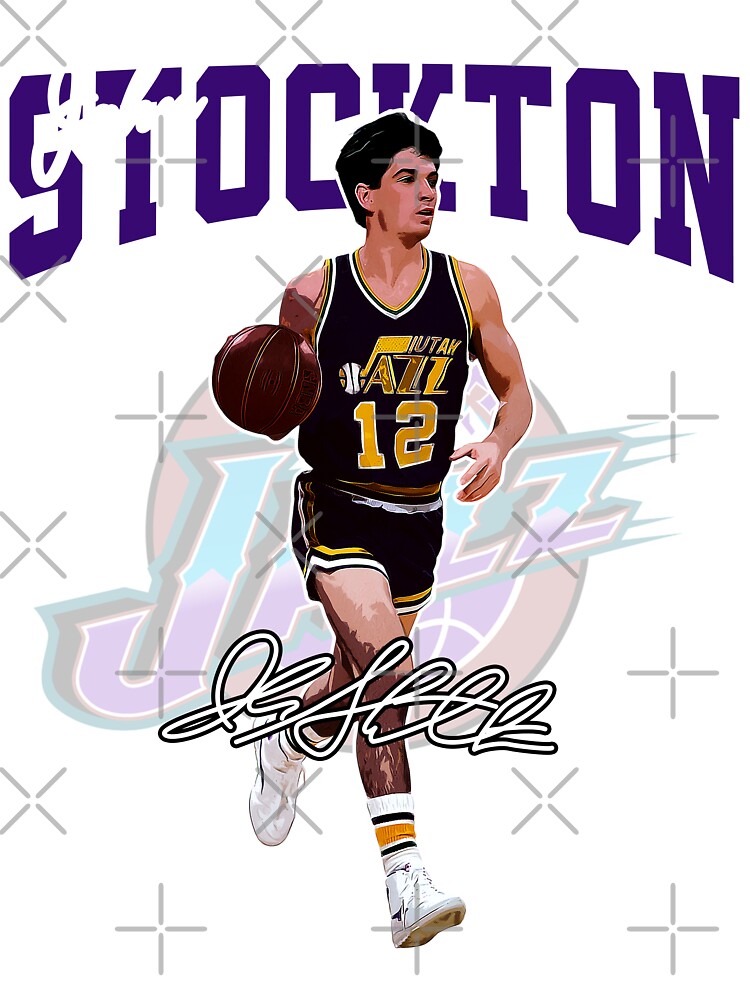The image is a detailed computer-generated depiction of a Utah Jazz basketball player, presumably John Stockton. The player is dynamically captured in motion, seemingly dribbling a basketball with his right hand. He is dressed in the team's black jersey and matching black shorts, both outlined with gold and white stripes. His jersey features the number 12 in yellow, and he wears white tube socks striped with black and yellow, accompanied by white basketball sneakers. The player's black hair adds to the lifelike detail of the image.

At the top of the image, the name "John Stockton" is prominently displayed, with "John" in a white handwritten style and "Stockton" in bold purple letters. This contrasts against the white-colored background, which is adorned with silver stars, plus marks, X’s, and crosses. Additionally, a ghostly rendition of the Utah Jazz logo, blending purple and turquoise, subtly occupies the center of the background, adding depth to the scene. The overall composition is rectangular, creating a visually striking tribute to the legendary basketball player.